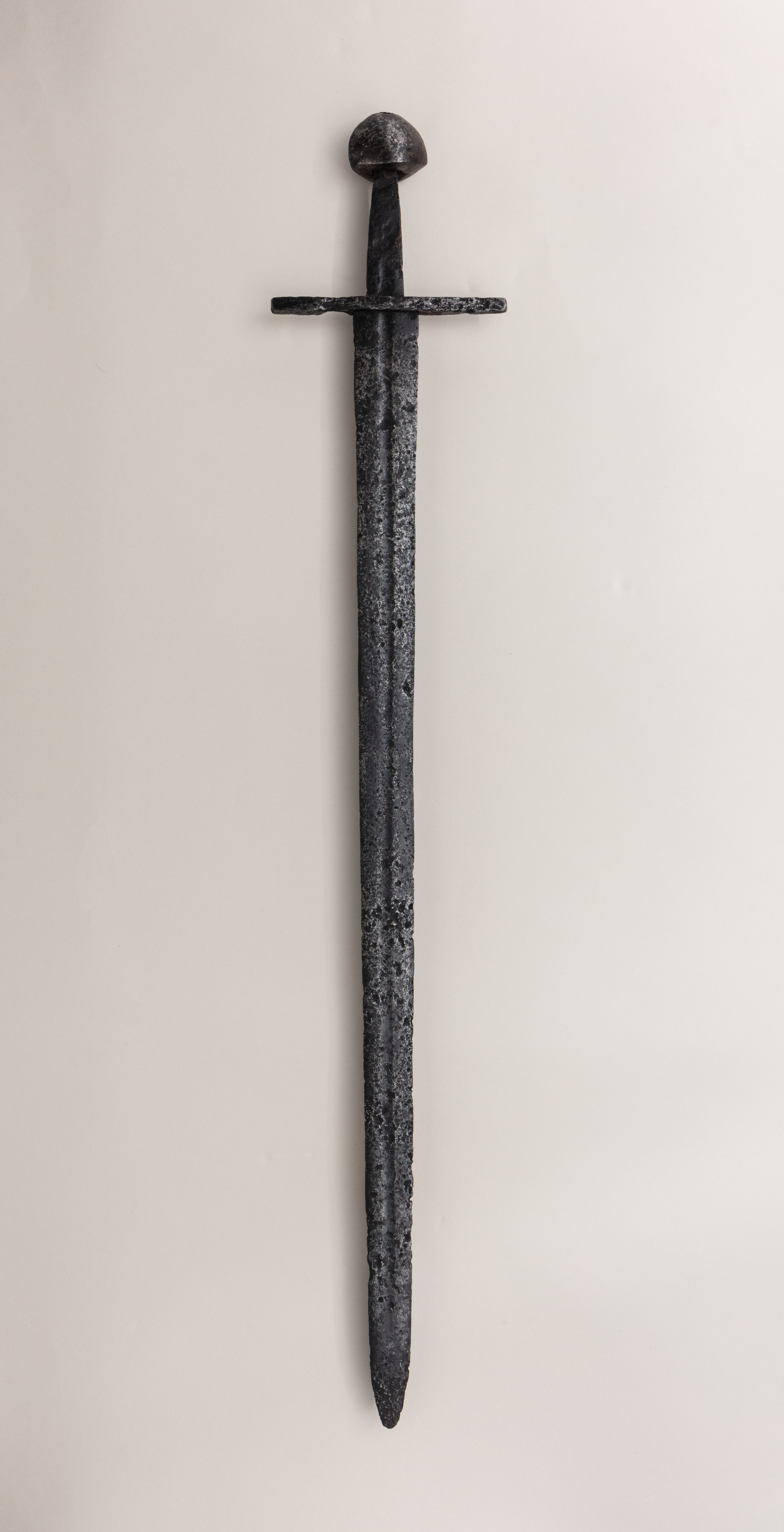The image showcases an ornamental and very dilapidated-looking sword hanging upside down on a plain, white wall. The sword, entirely made of metal, appears incredibly shabby and worn, with numerous dings and chips throughout its structure. Starting from the top, the pommel is misshapen, almost as if it weren't forged in a perfect circle or has been deformed over time. The grip, only a few inches long, is in relatively good condition. The crossguard, forming a classic T-shape, follows the trend of being dinged and slightly misshapen.

The blade, extending from the crossguard, exhibits a rough, stone-like texture with visible divots and pores, suggesting it might be of considerable age or made from an unusual material. The metal of the blade displays a variation in color, with the area near the hilt remaining dark and the edges taking on a grayish-silver hue, possibly due to patina. Towards the tip, the blade is indented and incredibly dull, culminating in a rounded point.

Overall, the sword appears to be around a foot and a half to two feet long, with a substantial portion of the photograph dominated by the lengthy blade. The wear and tear on the blade, including notches and marks, indicate it might have been used in combat or another significant event, and it could have historical significance, perhaps passed down through generations or discovered at an archaeological site.